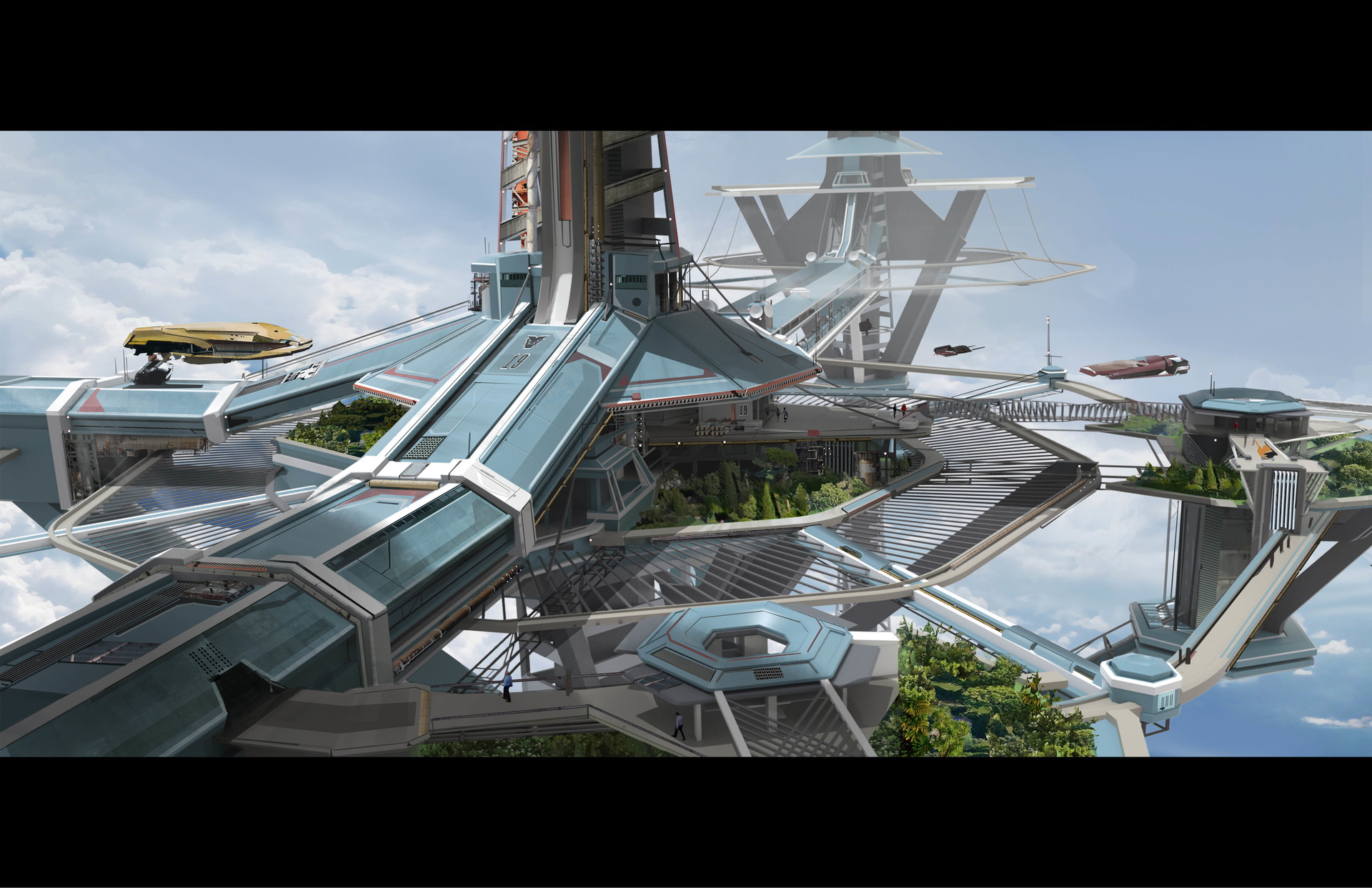This image is a detailed digital illustration of a futuristic hover city built high in the sky. The city features a large, blue, ship-like structure with multiple parts and levels, interconnected by tunnel-like pathways. The architecture has elements of advanced technology and steampunk aesthetics. This aerial metropolis includes elevated green gardenscapes with trees and bushes, creating an open, park-like environment. Various hovercrafts and spacecrafts, resembling metro trains, are seen parked or flying nearby. People can be seen walking along the decks, highlighting the bustling, yet serene life within this advanced sky city. White clouds surround the structure, emphasizing its lofty elevation.